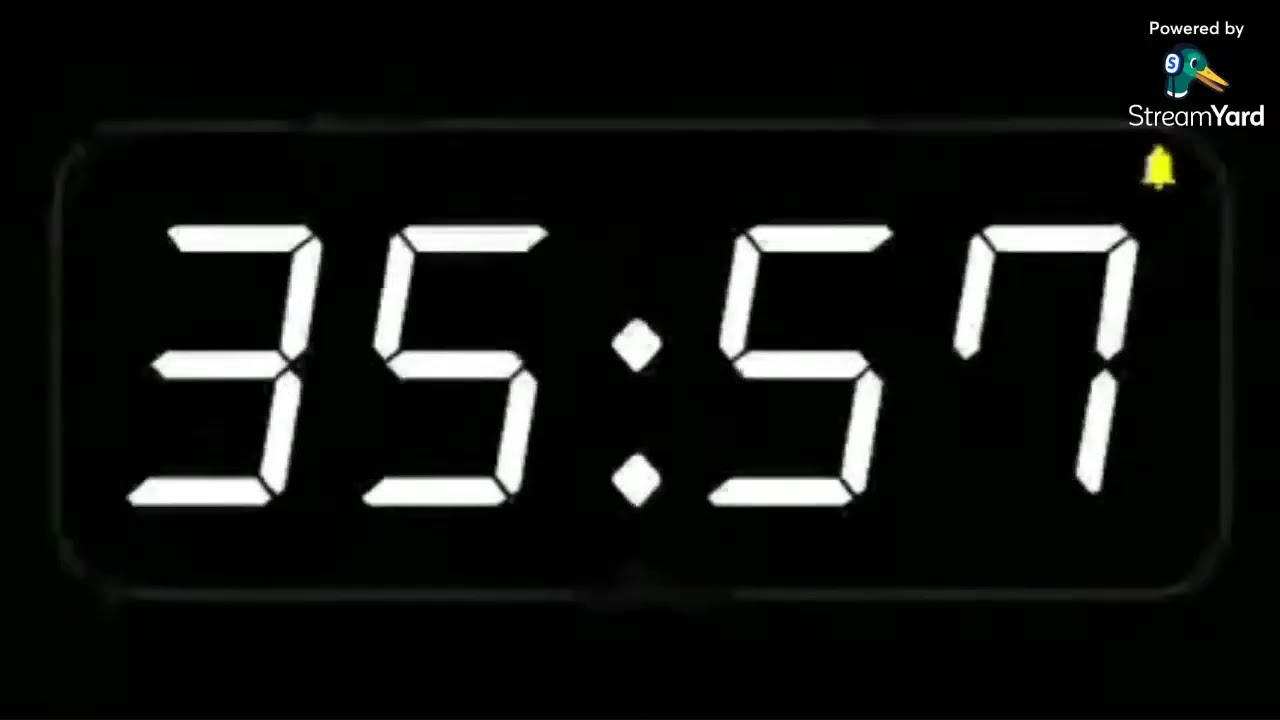The image in question features a digital clock display against a black background, with the time shown as "35:57" in traditional segmented white digits reminiscent of classic alarm clocks. Encircling the time display is a faint light gray rectangle with rounded edges. In the top right corner, there is a logo consisting of a green duck head with a gold-orange beak and black eyes, wearing a white headset adorned with the letter "S." The text "powered by StreamYard" appears beneath the duck image, accompanied by a small yellow bell icon. The overall design suggests a digital creation with a retro alarm clock aesthetic.